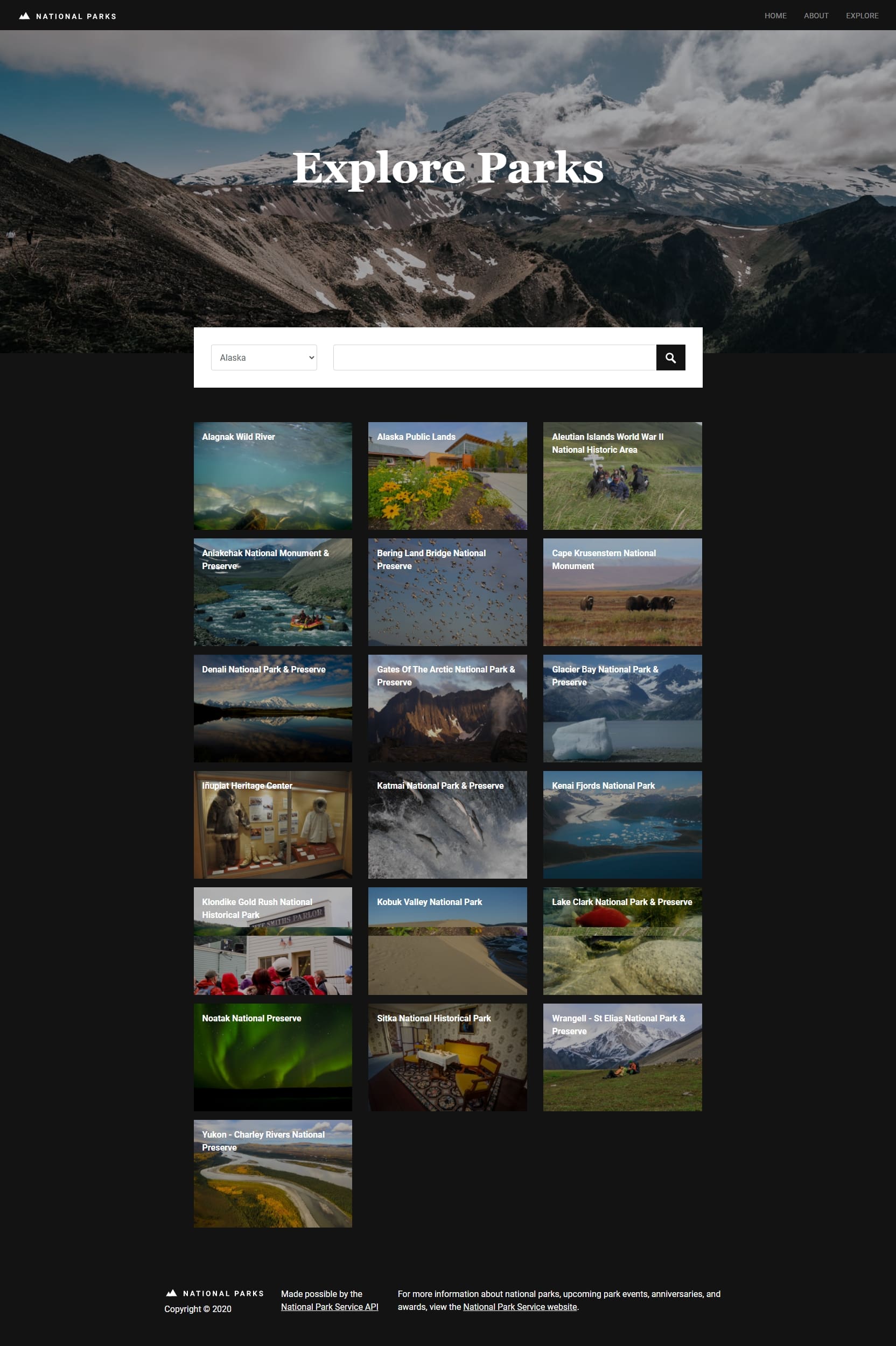The image features a webpage dedicated to National Parks. The header is a small black strip containing white text and an icon depicting a mountain, accompanied by the words "National Parks." The background showcases a stunning landscape with several mountains, a striking blue sky peeking out towards the left, and billowing clouds surrounding the peaks. 

Prominently positioned at the top center in bold, white Georgia font, the title "Explore Parks" stands out. Beneath this title, a white rectangular search bar is displayed. The search bar includes a dropdown menu on the left side where a state can be selected, with Alaska currently chosen, presumably because it is listed in alphabetical order. Adjacent to this is a query input field, followed by a small black square containing a white magnifying glass icon, tilted towards the upper left, indicating the search function.

Below the search bar, a series of images appear, representing various National Parks. The first image's text partially reads "Wild River," followed by others titled "Alaska Public Lands," "Alaskan Islands," and "World War II National Historic Area." This section includes visually captivating photos such as a person white water rafting on a body of water, a flock of birds, wild buffalo, a sunset over a body of water, and more scenic mountain landscapes. Additionally, a picturesque scenery filled with clouds is featured towards the right. The collection of images and details vividly captures the diverse beauty and adventure found within National Parks.